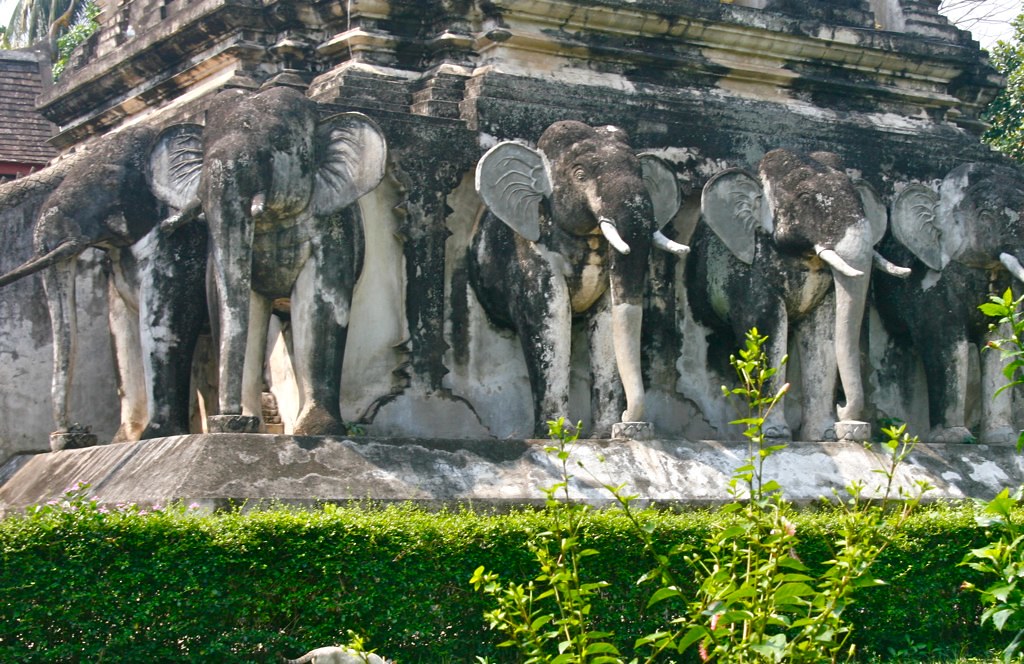In this outdoor photograph, a large, decorative building or monument serves as the focal point. Prominently featured are five impressive sculptures of elephants, crafted to appear as though they are emerging from the stone facade. Each elephant, meticulously carved and chiseled by either machine or hand, displays only its head, trunk, ears, chest, and upper limbs, which lend a strikingly lifelike quality. These sculptures are predominantly gray, with black spots indicative of weathering, possibly from water damage, giving the stone a mottled appearance. The structure itself is substantial and rectangular, adorned with elaborate carvings. Surrounding the base of this building are vivid green hedges and some colorful flowers, enhancing the contrast between the natural greenery and the architectural monument. Sunlight bathes the scene, casting reflections on the building and highlighting the intricate details of the weathered carvings.